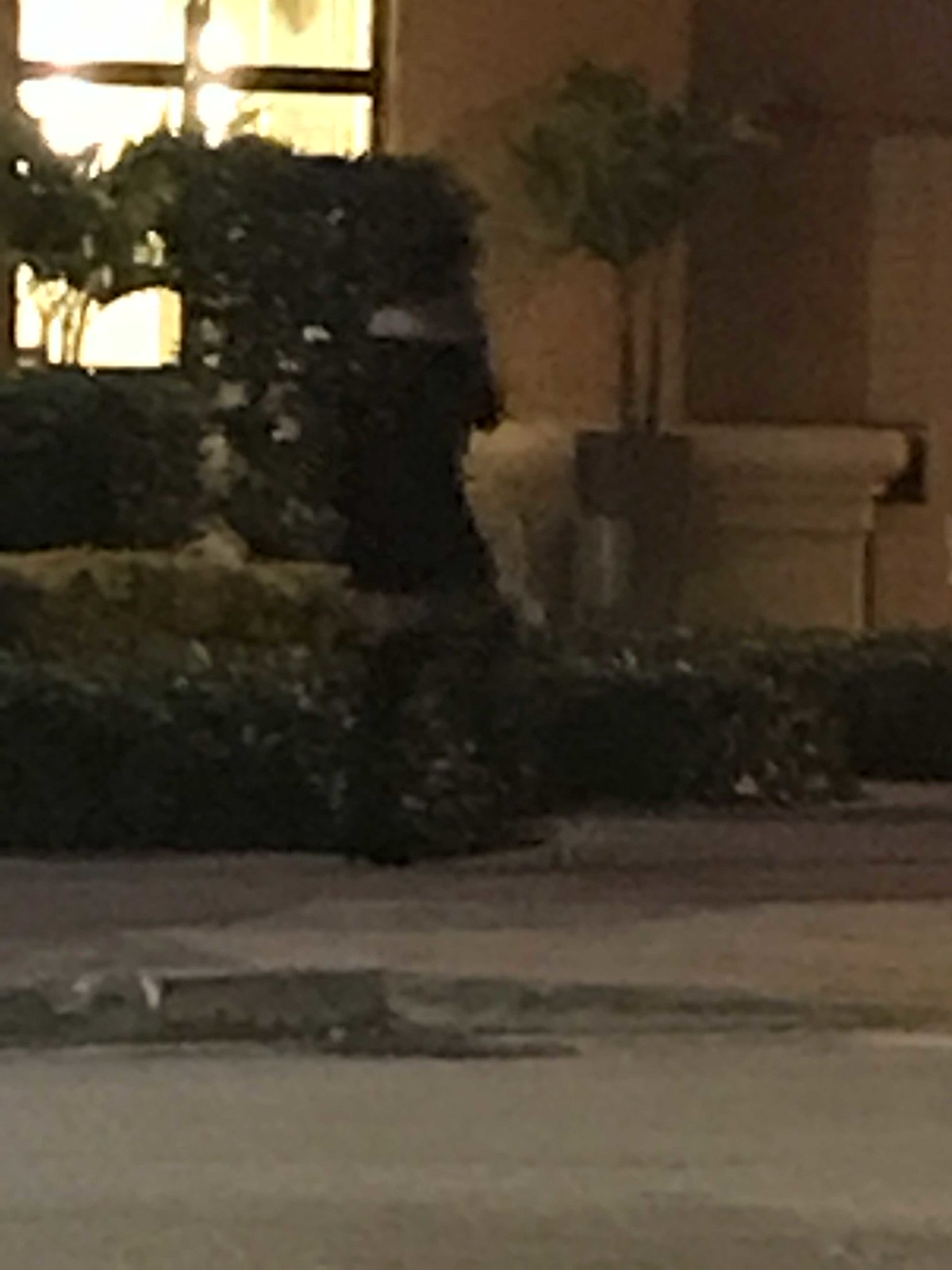This nighttime image, though blurry, captures a residential scene. An illuminated window occupies the top left corner of the photo, indicating someone is present inside the house with the lights on. In front of the house, there are bushes that add to the foliage. At the center of the image, slightly in the background, there's a potted plant resembling a small palm tree. The foreground features a gray-colored road with a visible curb, followed by a sidewalk lined with more plants, creating the impression of a front yard garden. On the top right side of the image, there's a cement column, possibly part of a facade, alongside either a door or a shadow resembling a door. The color palette is muted due to the night setting, dominated by shadowy hues of dark green, tan, and gray, giving the image a somber, indistinct quality.